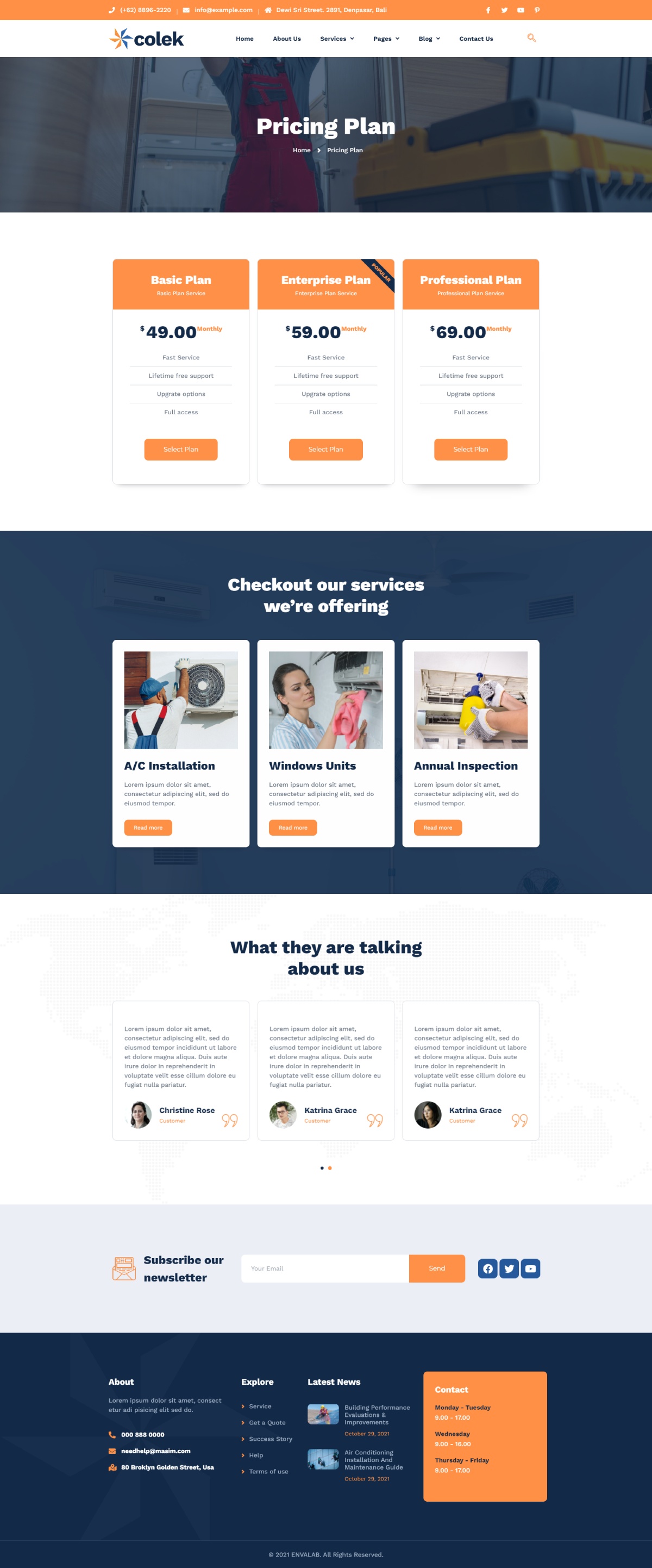This is a detailed description of the pricing plan page of Colek's mobile app website:

At the top of the page, there is an orange navigation bar featuring several options, which are too small to be legible. Directly beneath it is a white navigation bar, also with small options, but it clearly displays the Colek logo on the left. The logo includes the brand name "Colek" with a pinwheel icon adjacent to it—orange on the left side and blue on the right side.

Below the navigation bars, the page title "Pricing Plan" is prominently displayed. The background features an image of a person standing in a train doorway holding a small box, adding a contextual backdrop to the content.

The pricing plans are presented in three categories: 
- "Basic Plan" is highlighted in an orange box with white text.
- Next to it is the "Enterprise Plan".
- Finally, the "Professional Plan" is listed.

The respective costs for these plans are $49, $59, and $69. Each plan is accompanied by a description, explaining what it includes. Under each plan's description, there's an orange button likely intended for users to select and subscribe to their chosen plan.

Further down, a section titled "Check Out Our Services" lists various offerings such as AC installation, window unit services, and aerial inspection. 

Following the services section, there's a testimonial portion titled "What They Are Talking About Us". This section displays three testimonials, complete with pictures and names of the individuals providing the feedback.

Towards the bottom of the page, there is an invitation to "Subscribe to Our Newsletter," where users can enter their email address and submit it.

Finally, the page concludes with a site map for easy navigation.